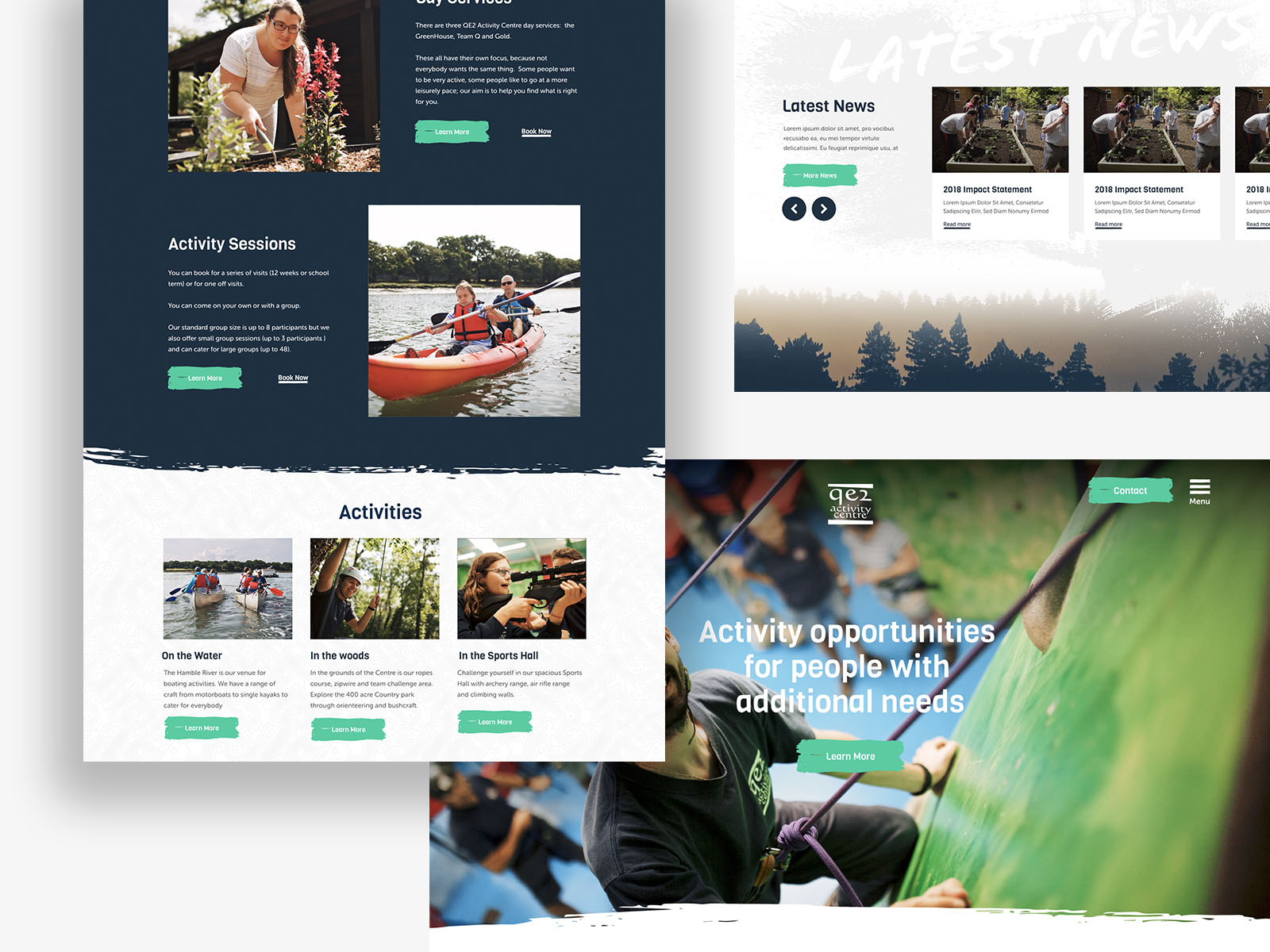This image is an artistic illustration depicting three sections of web pages arranged in a creative layout. 

The left section displays a vertically oriented web page featuring two prominent photographs. The first image shows a woman engaged in gardening, while the second captures a serene scene of two individuals canoeing on a lake. Accompanying these photographs are green "Learn More" buttons. Titled "Activity Sessions," this section outlines various activities. Below this header, the word "Activities" introduces three additional smaller photographs showcasing people participating in diverse activities: one on the water, another in the woods, and a third in a sports hall.

The upper right section, separated by a gray border, is dedicated to "Latest News." This segment also contains a green button and prominently displays two photographs of individuals gardening. The backdrop features a simple illustration of a tree against a skyline. The "Latest News" title is elegantly presented in white, fancy text at the top.

The bottom section depicts a horizontally oriented web page with a striking photograph of a person rock climbing or scaling an indoor climbing wall. The individual is secured with a rope around their waist. Centered in white text, the caption reads "Activity Opportunities for People with Additional Needs." This section also includes two green buttons, along with a menu button located in the upper right-hand corner of the image.